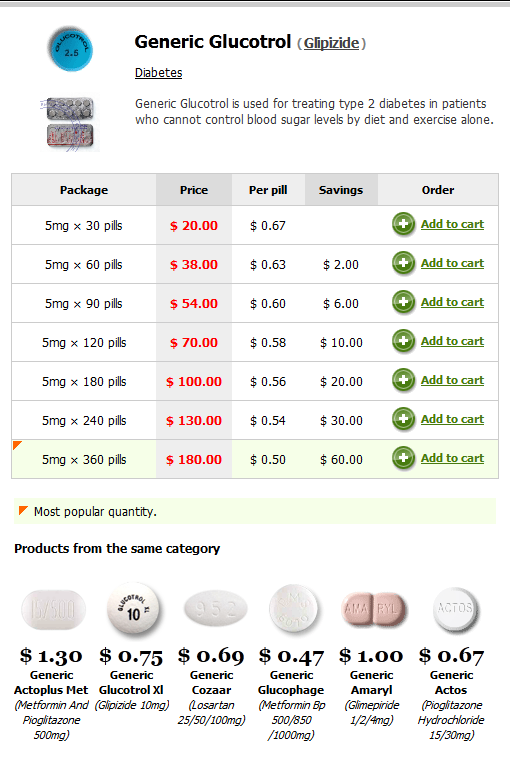The image is a screenshot of information pertaining to the generic medication Glucotrol, also known as glipizide. It features a link to additional diabetes resources. The accompanying text explains that generic Glucotrol is utilized for managing type 2 diabetes in patients who cannot control their blood sugar levels through diet and exercise alone. It is available in pill form.

Below the descriptive text, there is a table detailing the various packaging options for the pills, ranging in quantity from 30 pills to 360 pills, all at a dosage of 5 milligrams. The pricing varies from $20 for a 30-pill package to $180 for a 360-pill package. This results in a per-pill cost ranging from approximately 67 cents to 50 cents, with the largest option offering the lowest per-pill price. 

The table also highlights the potential savings for bulk purchases. Each row in the table features a green "Add to Cart" button for easy purchasing. 

Further down, the image notes that the most popular quantity among buyers is the 360-pill package. It also lists similar products, including generic Octoplasmet, generic Glucotrol XL, generic Cozaar, generic Glucophage, generic Amaryl, and generic Actos.